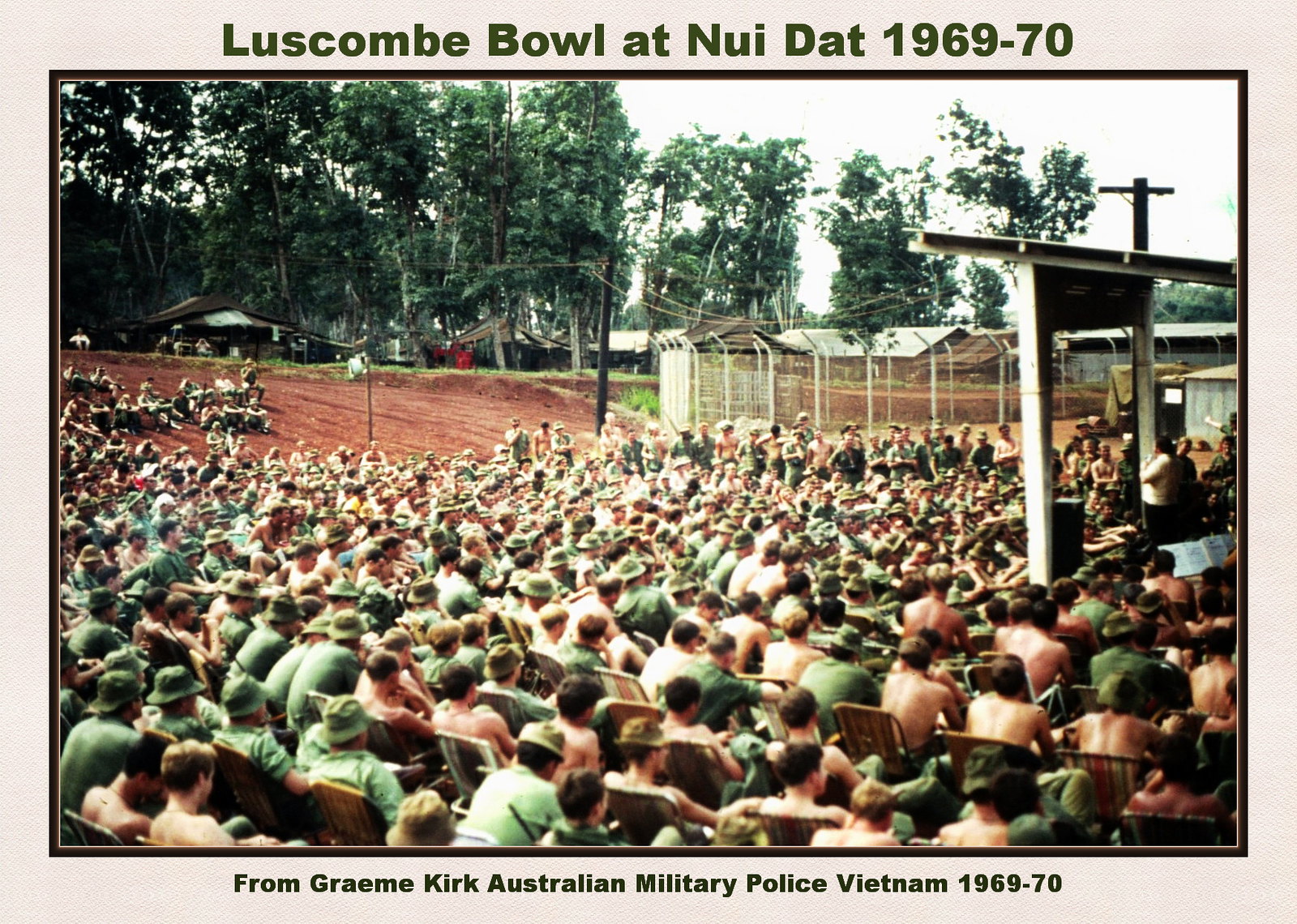This vintage photograph captures a large assembly of soldiers during the Vietnam War, specifically at Nui Dat between 1969 and 1970. The scene is teeming with hundreds of servicemen, some in green uniforms and others shirtless, lounging in beach or lawn chairs. They are gathered in an open field in what appears to be a forested area, signaled by the greenery and large trees in the background. The soldiers are fixated on a small stage to the right of the image, where a couple of individuals are either speaking or presenting, likely providing entertainment or giving a speech. The backdrop includes various buildings and tents, indicative of military barracks. The photo is bordered with text at the top and bottom reading, "Luce Combe Bowl at Nui Dat 1969-70 from Graham Kirk, Australian Military Police, Vietnam 1969-70," clearly marking the event’s era and location.